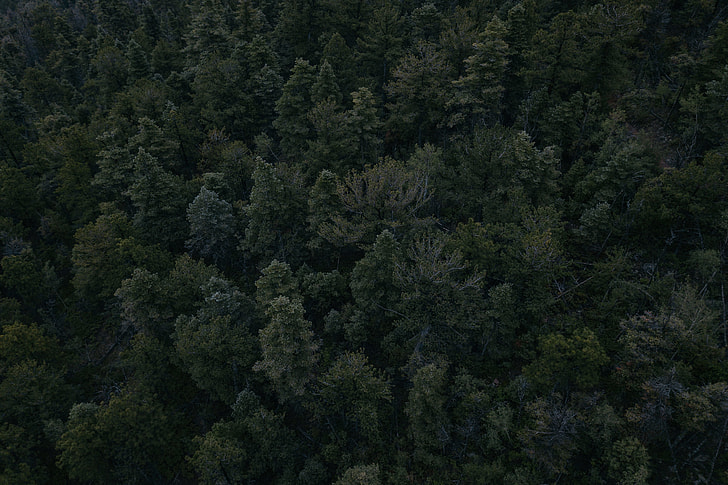This image offers a stunning aerial view taken from an airplane or helicopter, capturing an expansive, dense forest comprised predominantly of evergreen and pine trees. The entirety of the frame is filled with these verdant trees, tightly packed together to the point where the ground is completely obscured. The foliage exhibits varying shades of green, dominated by a rich forest green with occasional lighter patches, which may be attributed to different species or branches. There are no gaps, no visible land, water, animals, or human presence—merely an uninterrupted canopy extending beneath. The array of treetops ranges from tall, pointed shapes reminiscent of Christmas trees to bushier forms, each contributing to the overall lush and compact composition of greenery. This image captures the pure essence of nature, exuding an almost postcard-perfect quality in its simplicity and beauty.